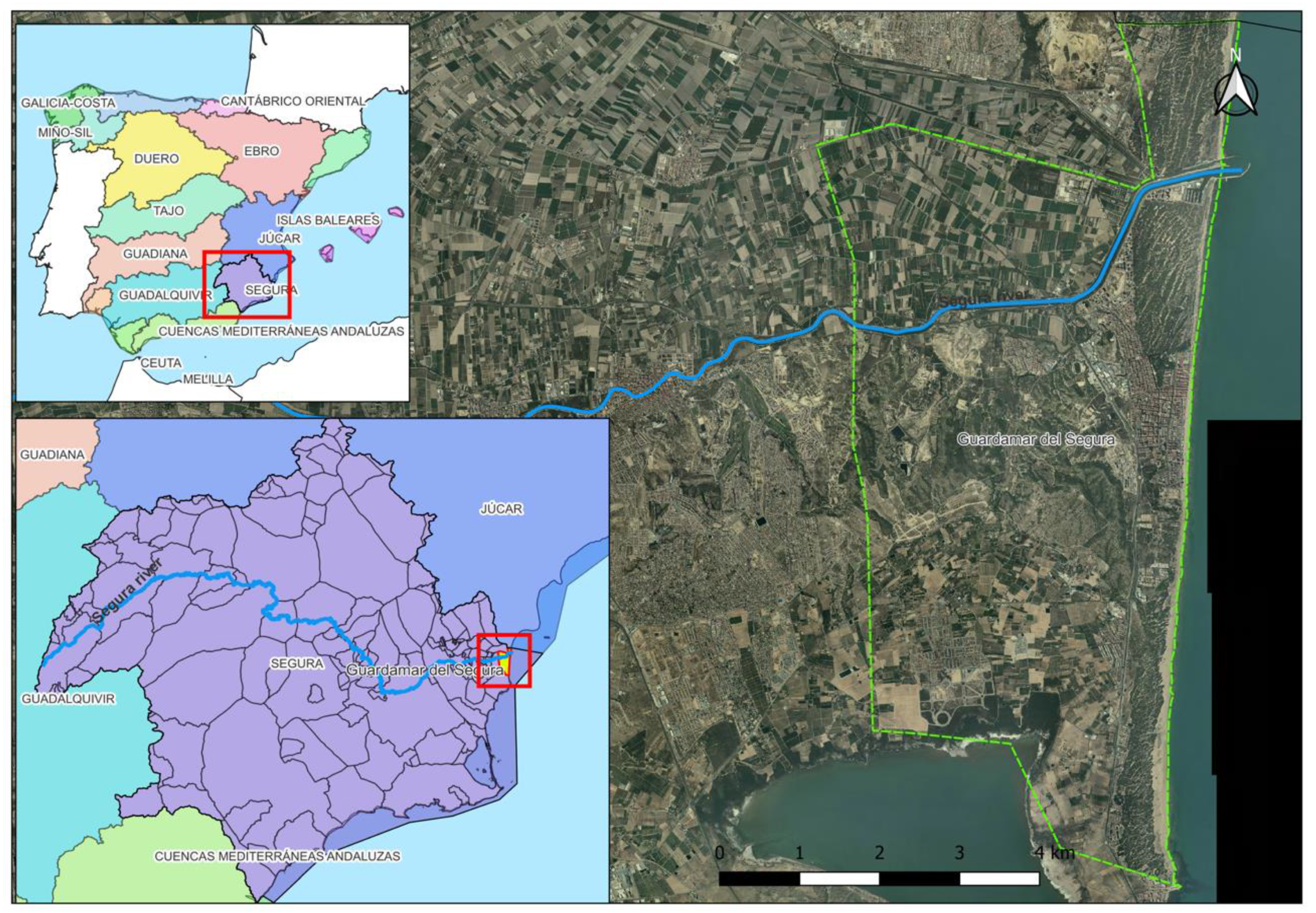The image is a detailed color infographic displaying three different maps of the same region. On the right side, there is a satellite view similar to Google Maps, featuring a blue line that winds from the middle to the top right corner, likely representing a river. Green perforated dotted lines zigzag towards the same or another destination. A black sidebar is present on the right side, with the place name "Guardamar del Segura" indicated.

On the left side, two smaller, colorful maps are overlaid at the top. The top-left map compartmentalizes parts of Spain into distinct color-coded sections: red for Duero, pink for Ebro, teal for Tajo (spelled T-A-J-O), and also shows Segura among other regions. These colors separate various geographical or administrative areas. Below this is another similarly styled map, where Segura is prominently displayed in purple.

The entire infographic gives a comprehensive visual representation of the location, with a scale indicating distances in kilometers, suggesting a span of the Mediterranean region likely involving Spain.